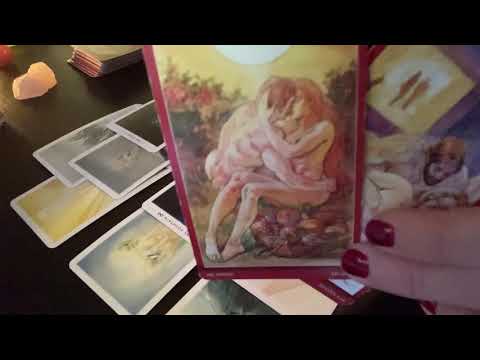A detailed image showcases a woman's hand with red nail polish on two fingers, delicately holding two tarot cards. The foreground card vividly depicts a naked man and woman embracing in a garden, with the woman seated on a rock, a yellow sun shining behind them, and lush foliage surrounding. The man has short brown hair, and the woman has long red hair. Another tarot card, partially obscured behind the first, shows a man with brown hair. Both cards are held over a black table scattered with pastel-colored tarot cards and a prominent pink crystal, giving the scene a mystical aura.